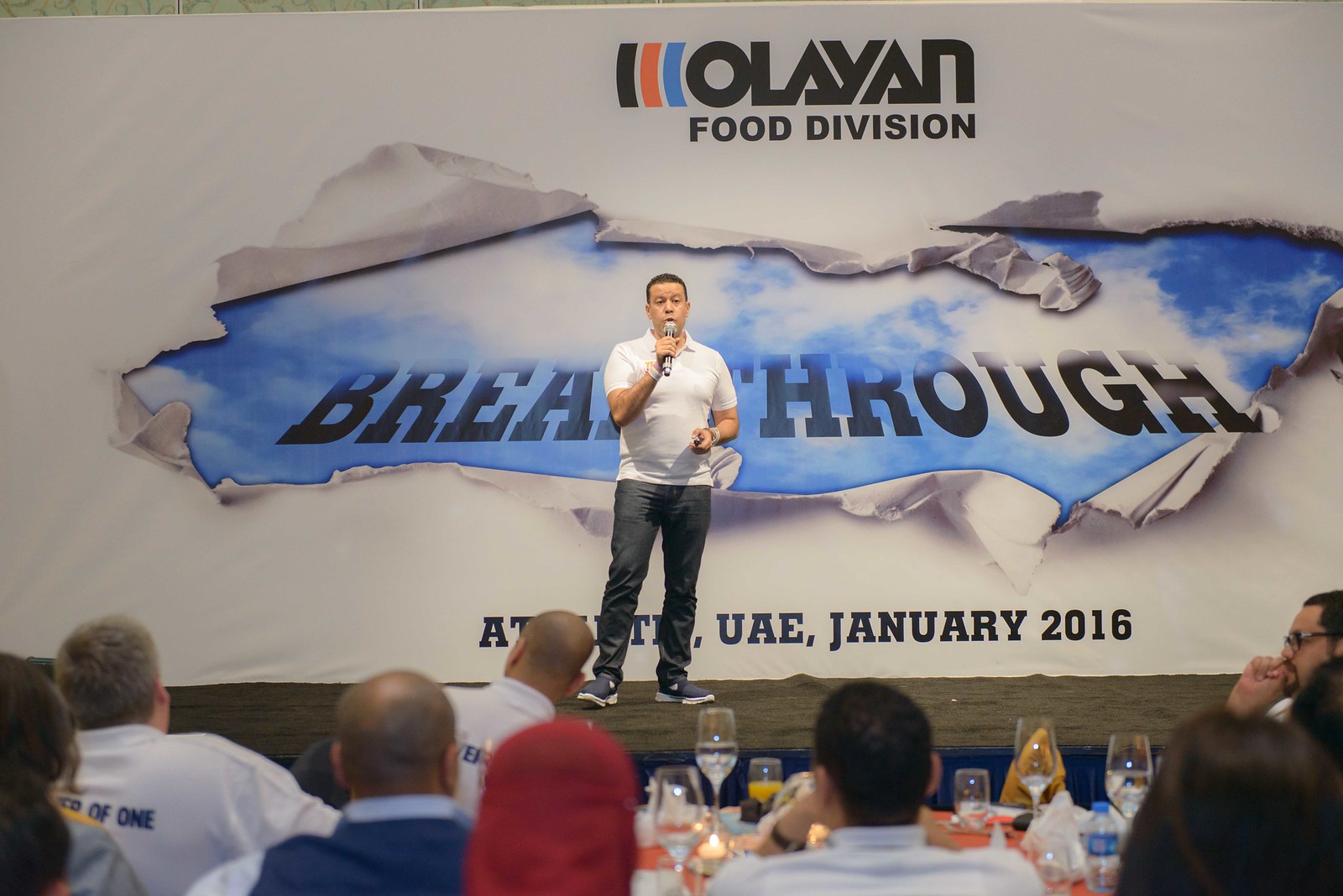The photograph captures a man giving a speech on a stage, wearing a white polo shirt, dark denim jeans, and blue shoes, while holding a microphone. He is addressing an audience seated at tables adorned with wine glasses and candles, predominantly male with a few women. The stage features a brown carpet and a striking backdrop, a large white wall with the top displaying the logo "Olean Food Division." Central to the backdrop is an image of a paper-like material being torn, revealing a blue sky with white clouds behind it and the bold black text "Breakthrough." Below this, the date and location, "AUE January 2016," are visible. The photograph is taken from the perspective of the audience, capturing the scene vividly.